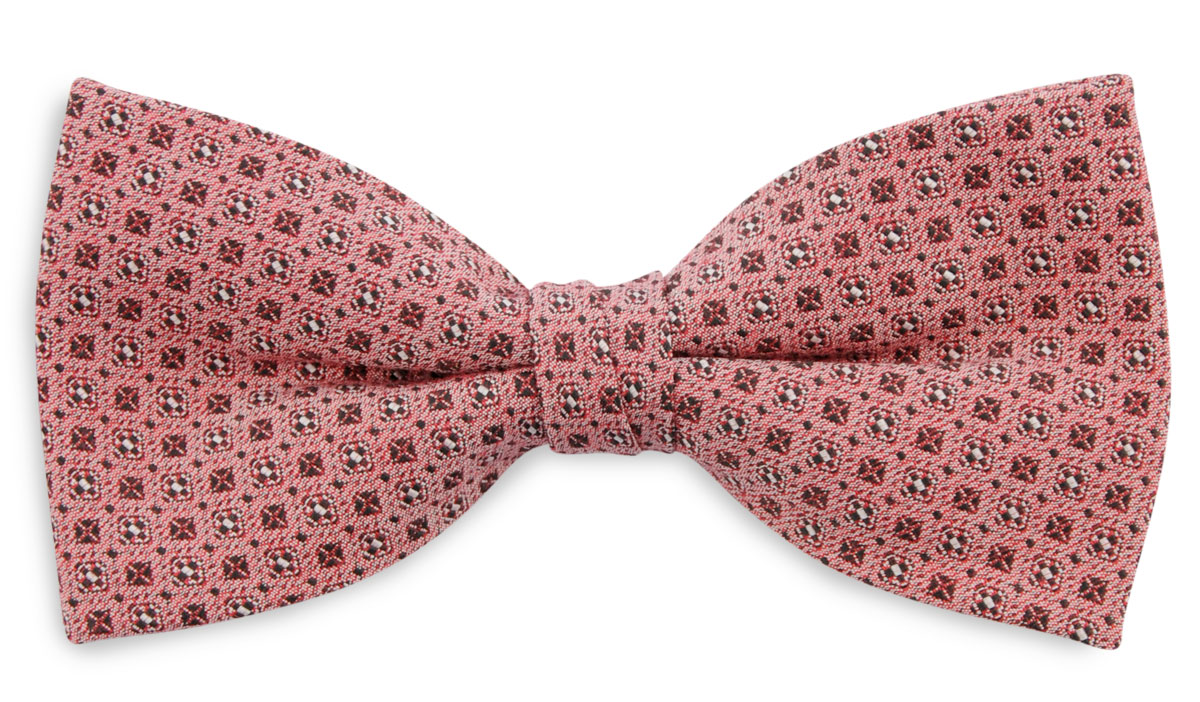The image is a close-up color photograph of a perfectly shaped bow tie against a white background, possibly photographed inside a light box. The bow tie is the sole focus of the photograph, showcasing its intricate design in great detail. The fabric of the bow tie is a rosy mauve or washed-out pink. The pattern on the bow tie consists of alternating small squares. Some squares have a black background with an X in the mauve color, while others resemble the top face of a dice showing the number four, arranged in white with dots. The pattern, which appears somewhat like a checkerboard, covers the entire bow tie, including the cinched middle section. The bow tie is likely a clip-on, inferred from how the fabric is arranged at the front.